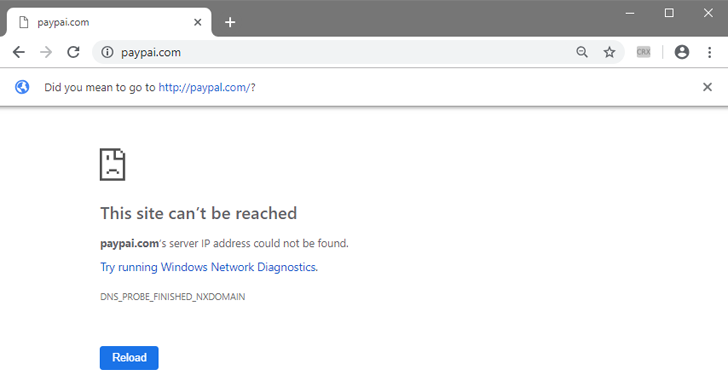The image depicts a web browser screen where the user appears to have attempted to navigate to PayPal’s website but inadvertently entered "paipai.com" instead of "paypal.com." 

At the top of the screen, in the web address bar, "paipai.com" is typed. The search bar is gray, and the incorrect URL is displayed in black text on a white background. To the right of the search bar, there is a search icon, followed by a star icon, a box labeled "crx," a small black circle symbolizing a user, and three vertical dots representing more options.

Below the search bar, a suggestion box appears on a white background. It states, "Did you mean to go to http://paypal.com?" written in blue text, accompanied by a black question mark.

Further down, there is a gray-outlined folder icon indicating an error alert. The message below it reads, "This site can’t be reached. paipai.com's server IP address could not be found." In blue text, it suggests, "Try running Windows Network Diagnostics." Additionally, a gray note at the bottom mentions "DNS_PROBE_FINISHED_NXDOMAIN," highlighting the specific error.

Finally, a blue "Reload" button is visible, encouraging the user to retry loading the page. The overall screen demonstrates the typical browser response to an incorrectly entered URL and offers relevant solutions and suggestions for the mistaken entry.